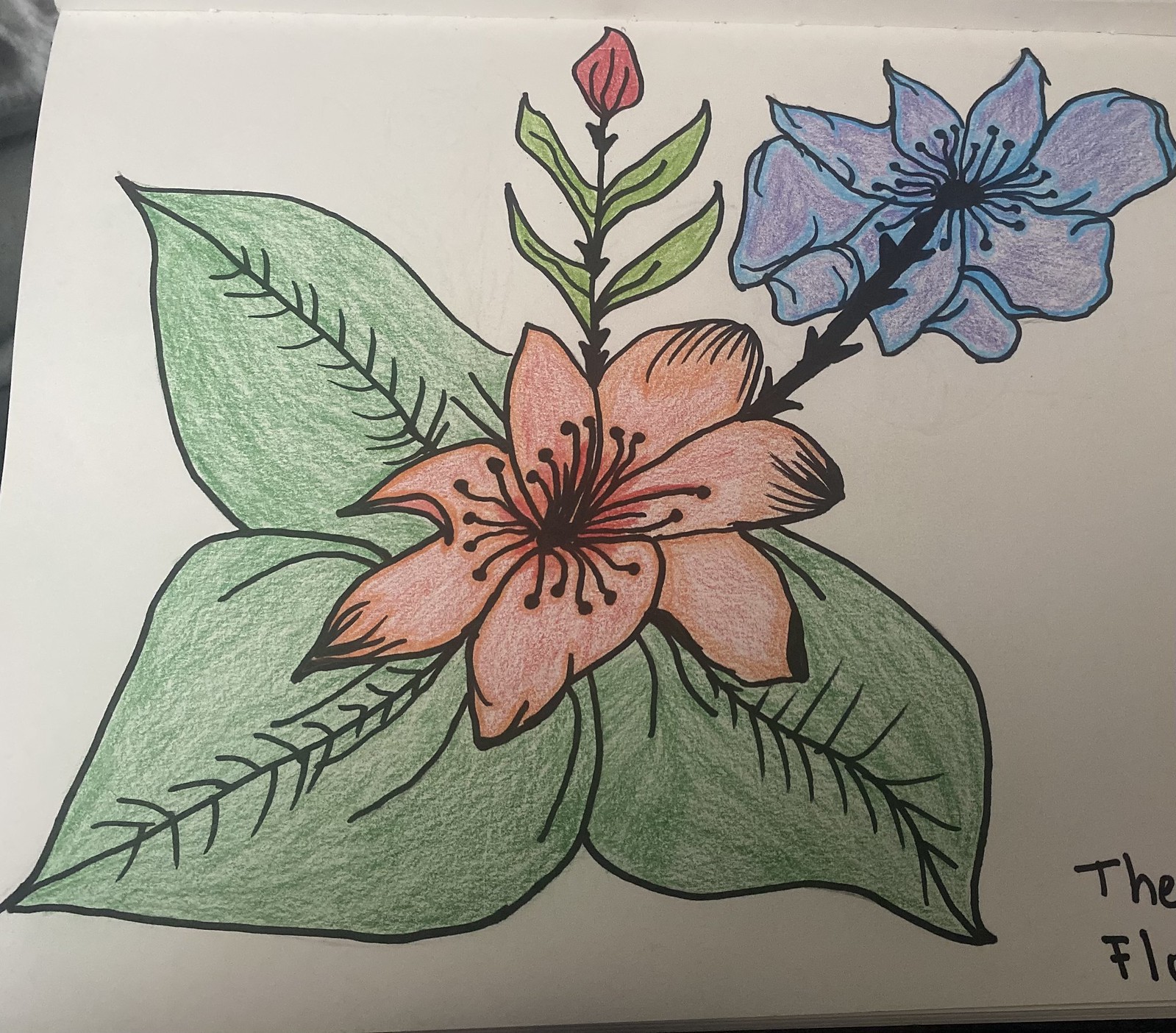An intricate and vibrant drawing depicts a collection of flowers, crafted using colored pencils or crayons to create a soft, matte texture. The composition, set against a plain white background, features bold, black line work that outlines the elements, likely rendered with a marker. In the bottom right-hand corner, partially visible letters spell out "T-H-E-F-L," hinting at a cut-off inscription.

The foreground showcases three prominent leaves, each defined by thick black edges and intricate vein patterns. One leaf extends to the left, another to the right, and the third diagonally towards the bottom left. A delicate pink flower, centrally located, is detailed with black lines representing the filaments. From its base, a black stem curves to the right, leading to a second flower in a gradient of purple and blue hues.

Adding to the layering of elements, a light yellowish-green leaf sits above, connected to a small red flower emerging from its top. This thoughtful arrangement of botanical elements exudes a sense of natural beauty and artistic detail.